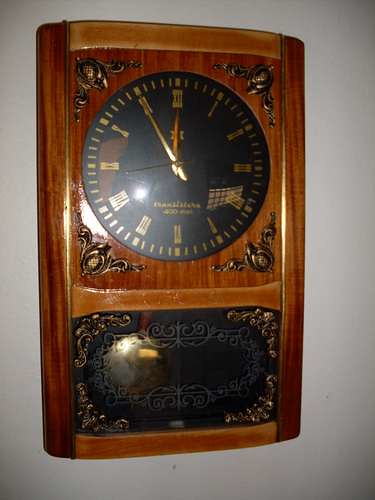The photograph depicts a beautifully crafted, antique-looking wooden wall clock with a gloss finish, characterized by its light and medium brown hues. The clock is rectangular, its longest side oriented vertically, and is divided into two main sections. The top section houses a standard black analog clock face adorned with gold Roman numerals, indicating a time of 11:55, and gold clock hands. The frame around the clock face features intricate gold embellishments in its corners. A reflection from the camera flash can be seen in the left bottom corner of the clock face, slightly blurring that area.

The lower section encases a swinging pendulum, which is visible through a pane of etched glass. The pendulum, positioned towards the left side of the clock, consists of a gold circle suspended by a red stick. Elegant gold decorations can also be found in the corners of this glass section. The clock's background is a simple white wall, highlighting the intricate details and wooden elegance of the timepiece.